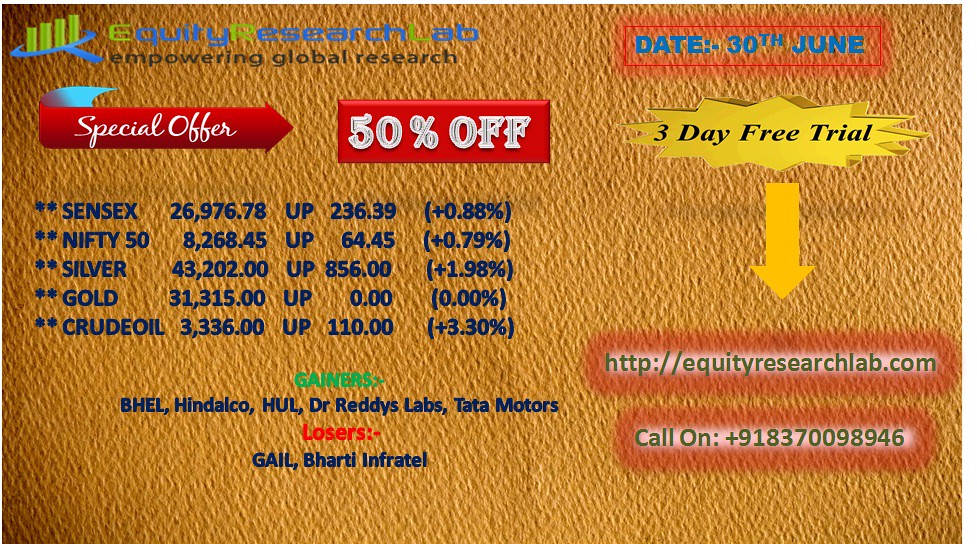The image is an advertisement for a financial analyst service with a visually cluttered layout on an orangish-yellow, textured background that resembles fabric. At the top, a logo reads "Equity Research Lab: Empowering Global Research," accompanied by a date, "30th June." Beneath this is a call-to-action section featuring a "Special Offer: 50% Off" and a "Three-Day Free Trial," highlighted by a large arrow pointing down to the website URL - "http://equityresearchlab.com" - and a contact phone number. 

The central area displays a list of investment options and their current market performance, including prominent indices like "SENSEX 26976.78 up 236.39 (0.88%)" and "NIFTY-FIFTY." There are also mentions of commodities such as "Silver, Gold, Crude Oil." Below these are various company names categorized by performance: gainers (e.g., "BHEL, HINDALCO, HUL, Dr. Reddy's Labs, Tata Motors") and losers (e.g., "GAIL, Barty, Infratel"). The overall text is difficult to read due to poor color contrast, with various shades of blue and green text atop the orange background, making it non-ADA compliant. The layout is scattered, offering a visually overwhelming and aesthetically unpleasing presentation.